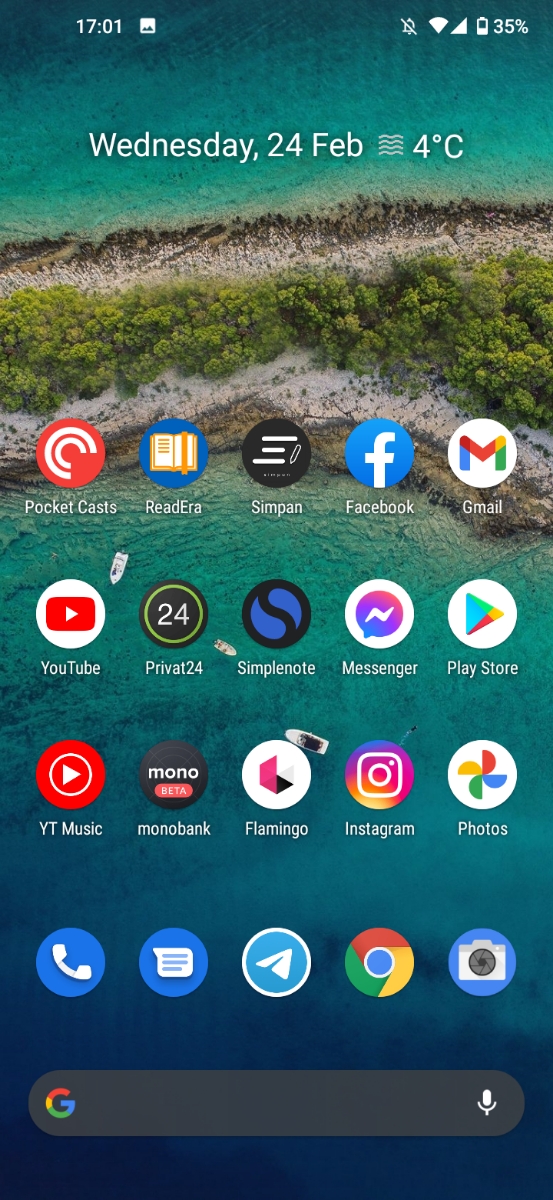A stunning aerial view of an uninhabited island captured on an iPhone, displaying a serene landscape. The island, bordered by clear turquoise waters on both sides, is narrow and filled with wild grasses and weeds scattered through its middle. The seaweed along the shores adds a touch of natural beauty to the scene. The iPhone screen shows essential details: a 35% battery life, full network connection, and silent mode activated. The time is prominently displayed at 17:01 and the date is Wednesday, February 24th with a chilly temperature of 4°C. The interface showcases various app icons including Pocket Casts, ReadEra, SimPAM, Facebook, Gmail, YouTube, Privat24, SimpleNote, Messenger, Play Store, YT Music, Monobank, Flamingo, Instagram, and Photos. The bottom row features Phone, Messages, the Internet, Google Chrome, and Camera apps enclosed in a blue circle. At the very bottom, a gray box with the Google "G" and a microphone icon is visible.